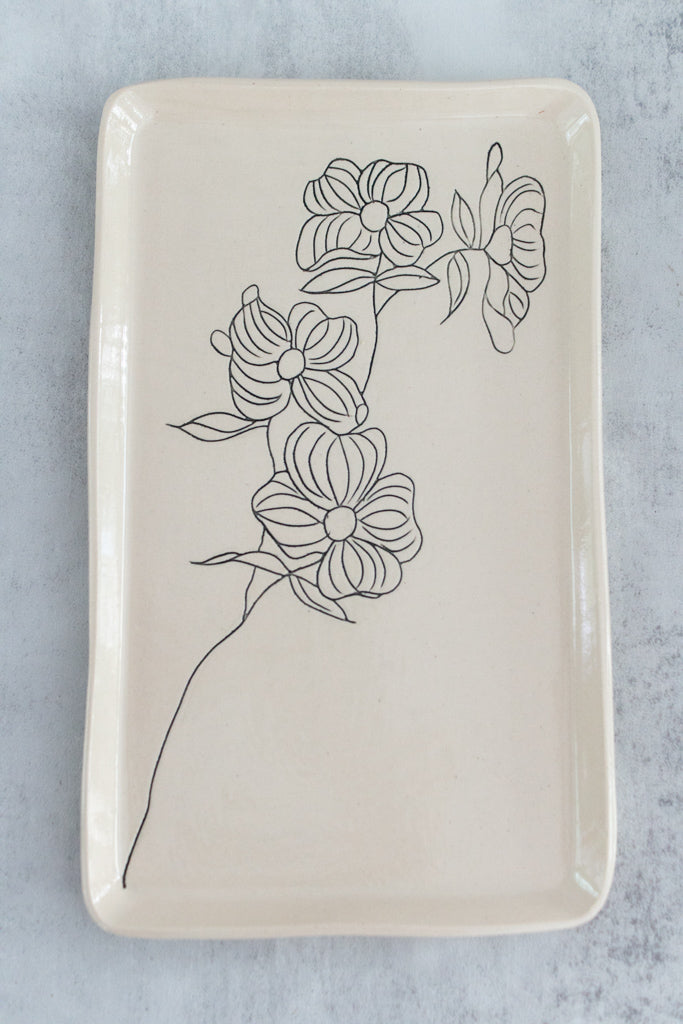The photograph features a large, rectangular serving plate made of shiny, ivory-colored ceramic. The plate, centered against a textured light gray background, showcases a detailed, monochromatic design of four delicate flowers, each with five petals and a couple of leaves. These flowers are interconnected along a single, continuous stem that extends diagonally from the bottom left corner to the top right corner of the plate. The design is etched into the ceramic in fine, thin lines, giving it an elegant, stencil-like appearance. The edges of the plate are slightly angled, adding to its polished, sophisticated look.